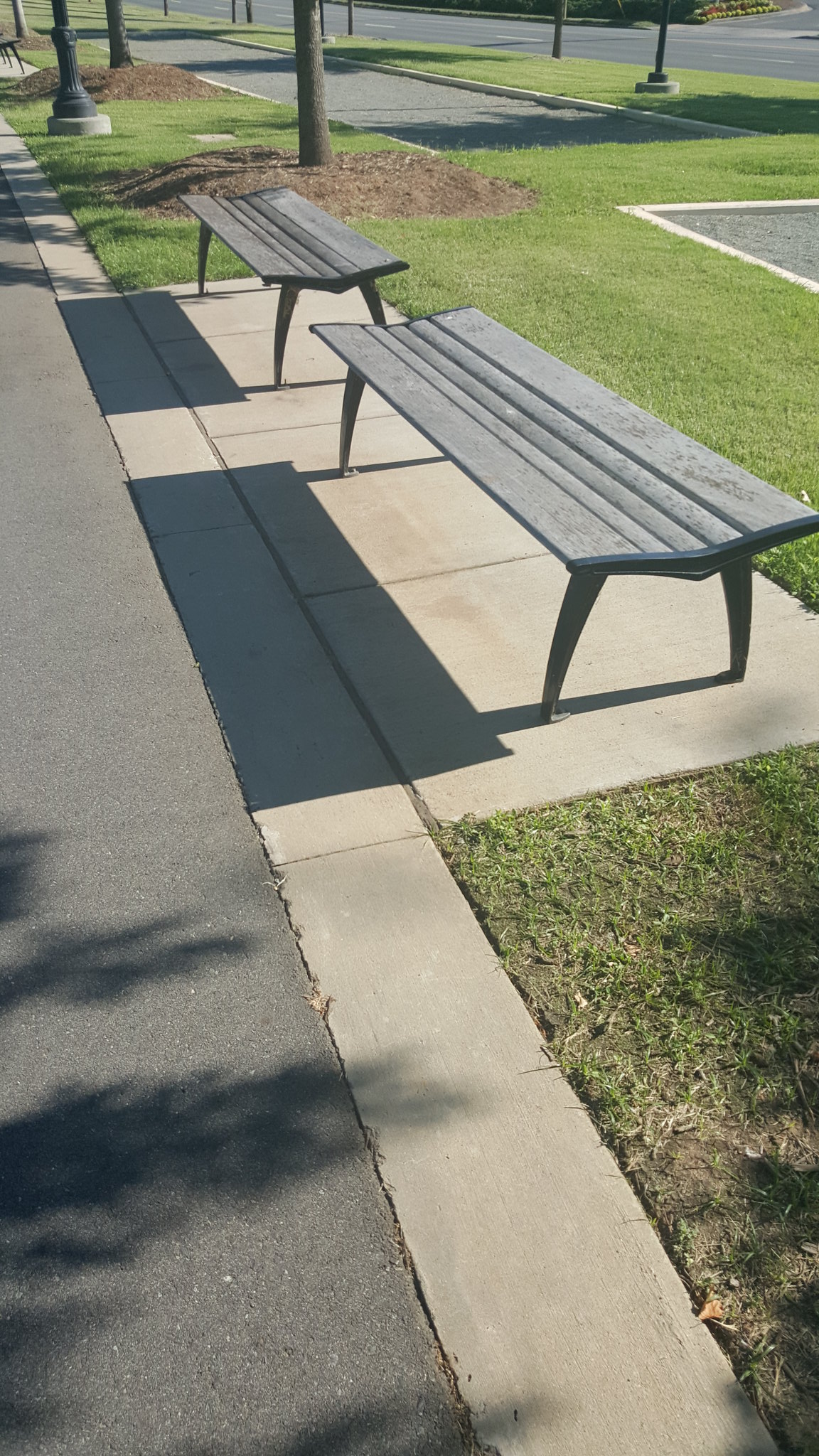The photograph captures a well-maintained, park-like setting dominated by two simple, backless park benches, positioned adjacent to each other on a clean, concrete slab. These benches, made from different boards of wood and colored gray, feature a slight valley dip for water drainage. The image is taken from a slight angle, creating a perspective that highlights the benches aligned parallel to a long tarmac path. A grassy verge borders the path, showcasing meticulously landscaped, vibrant green grass. In the background, a tree surrounded by mulch stands on a small mound of earth. The scene is bathed in sunlight, casting distinct shadows of the benches onto the concrete floor, accentuating the bright and clear atmosphere. The background includes hints of lampposts and what appears to be a street, suggesting the proximity to an urban area. The entire area is impeccably clean, with no visible debris or litter, further emphasizing the park's pristine condition.